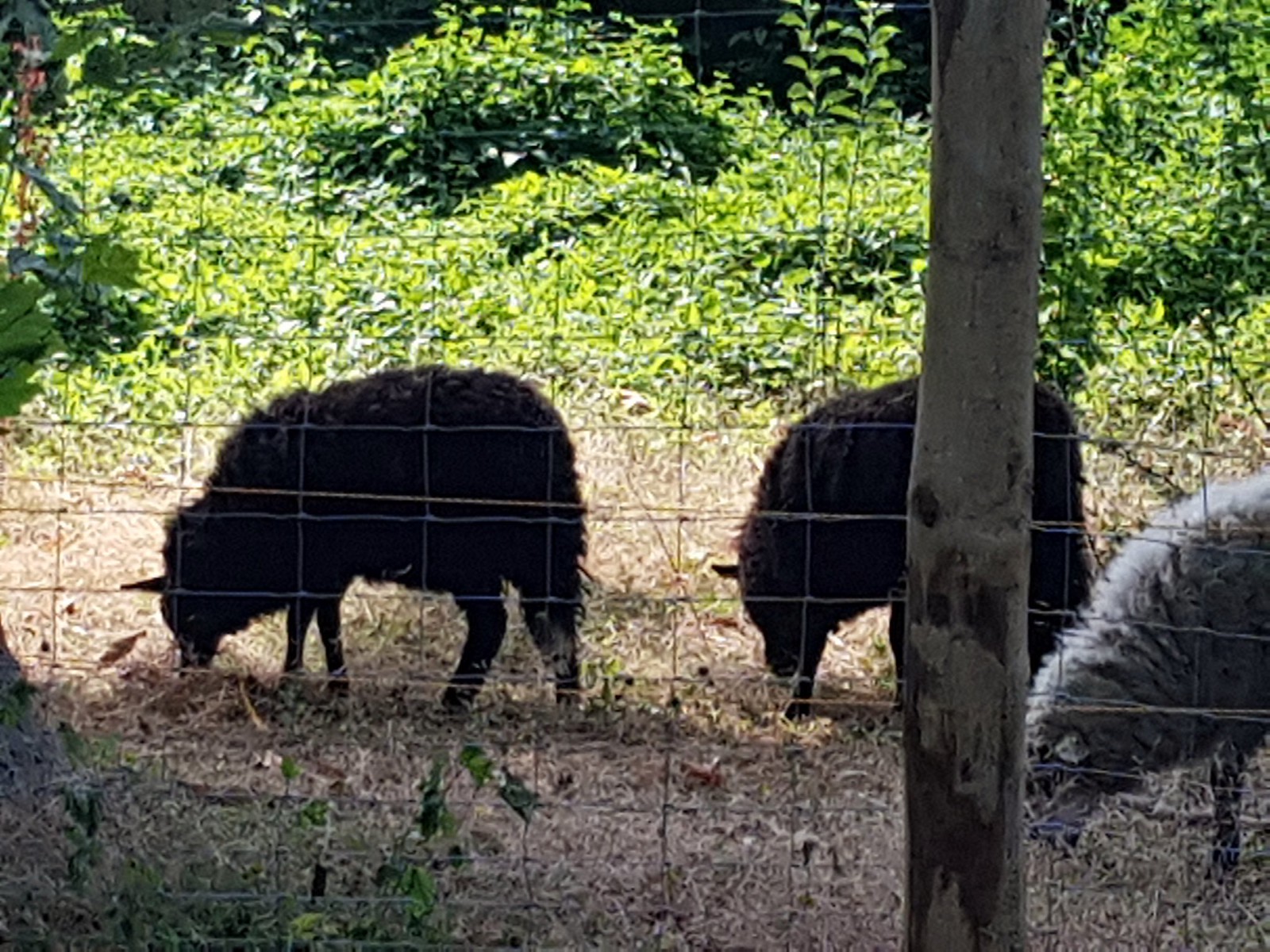The photograph features three sheep—two black and one grey—situated behind a white enclosure in a grassy paddock. The sheep are engaged in grazing, with their heads bent toward the dry, light-colored grass that appears dead in patches. A tree trunk in the foreground slightly obscures the middle black sheep. The lush green shrubs and foliage in the background contrast with the arid ground, underlining the bright, sunny conditions of the day. The enclosure fence is white and thin, possibly attached to wooden posts visible on the right-hand side of the image.